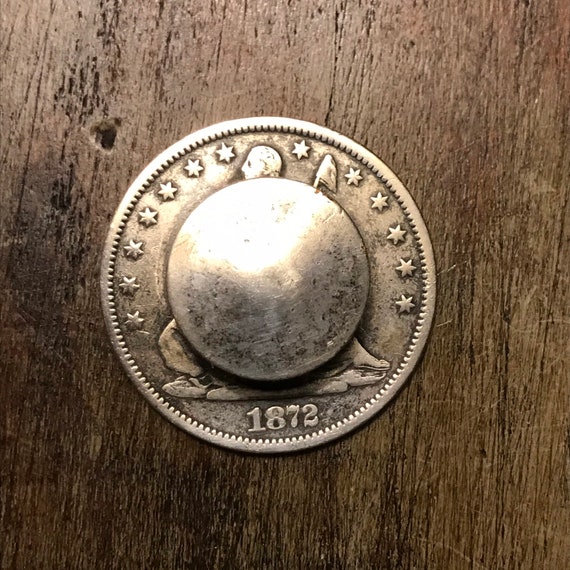The image features a seemingly silver coin resting on a dark brown wooden surface, which bears noticeable scratch marks and a hole in the upper left-hand corner. The wood grain runs vertically along the surface. The coin itself displays a smooth outer edge, transitioning to a ridged pattern encircling its interior. The top half of the coin is adorned with a series of six-pointed stars, while the bottom clearly shows the date "1872." 

In the center of the coin, a prominent blank circular dome obscures part of an intricate design beneath. Visible from behind this dome is the head of a man looking to the left. The man appears to be involved in a flag-planting action, suggested by elements that resemble a flag and possibly a ground or base. The coin, which seems worn and slightly dirty, is more illuminated on the top half, casting a shadow on the lower portion. This lighting effect hints at a textured and aged appearance, particularly given the discolored, goldish-silver tint described.